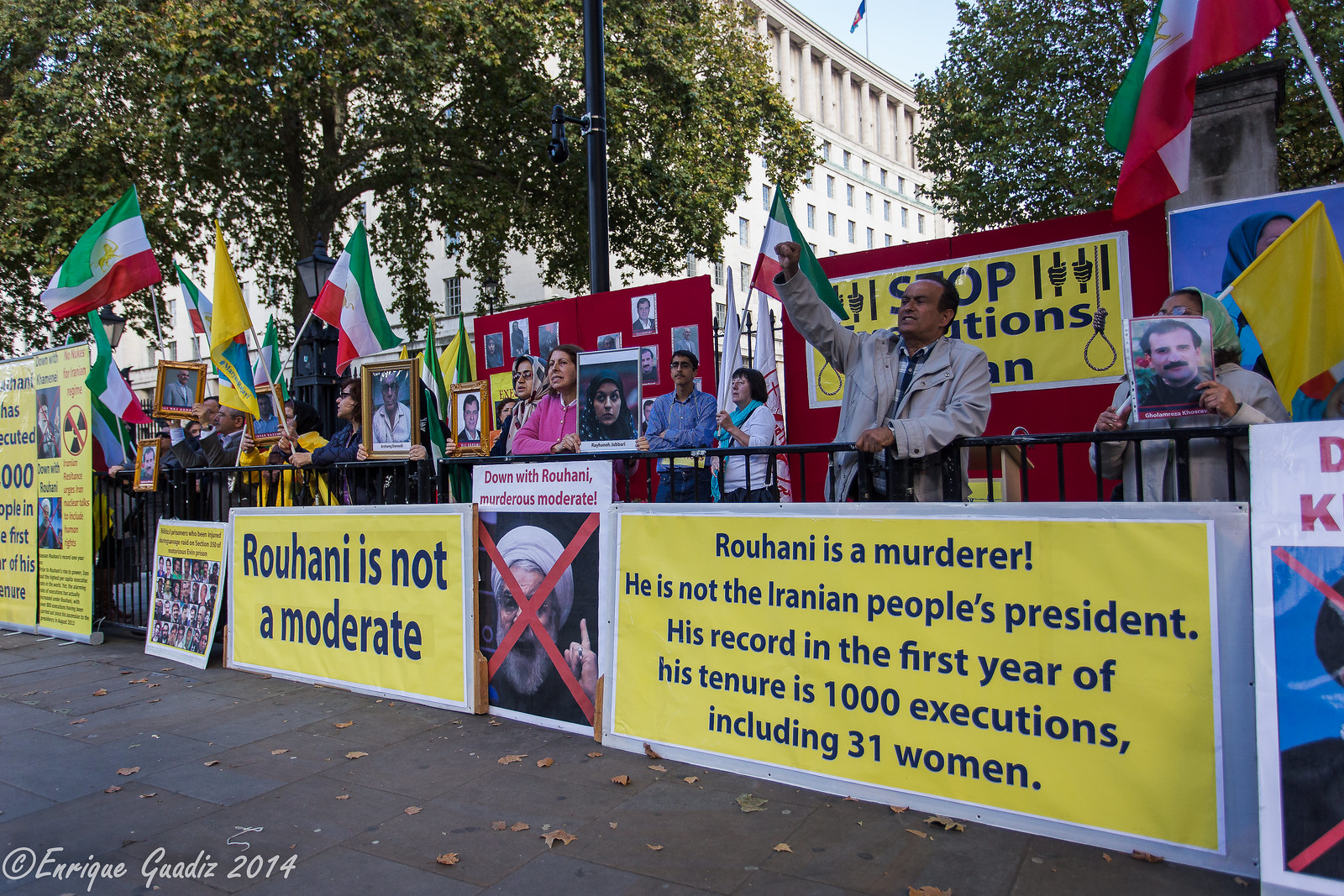In the foreground of the photograph, a line of approximately 20 protesters is gathered behind metal railings on a street or sidewalk. They hold up various signs and framed portraits, predominantly of young men. Dominating the scene are large yellow signs with bold, dark lettering, some of which read "Rouhani is not a moderate" and "Rouhani is a murderer. He is not the Iranian people's president. His record in the first year of his tenure is 1,000 executions including 31 women." A prominent image of Hassan Rouhani with a red X through his face features on these signs, accompanied by the phrase "Down with Rouhani, murderous moderate."

Several protesters wave flags in red, white, and green stripes, likely Iranian flags, alongside a flag with red, blue, and yellow colors and noticeable yellow trim. Additionally, a sign depicting a noose and the word "STOP" can be seen amidst the crowd.

Behind the protesters, a large building looms in the background, with several trees and a light pole visible nearby. The sky is clear, suggesting the photo was taken during the daytime. The bottom left corner of the photograph is marked with the copyright "Enrique Gladys, 2014."